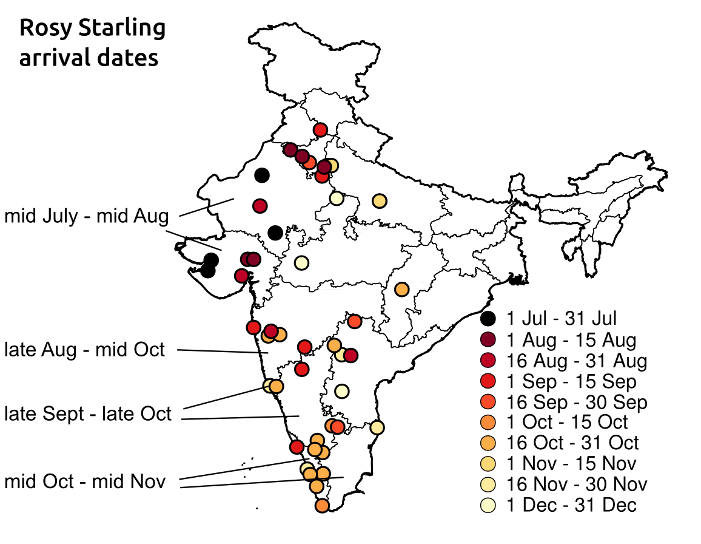The image is a detailed black and white map of India, prominently titled "Rosy Starling Arrival Dates" at the top right corner. The map is dotted with various color-coded dates indicating the arrival periods of rosy starlings, spanning from July to December. There are dark blue dots representing the period from July 1st to July 31st, with subsequent dots in shades of purple, red, orange, and yellow marking bi-monthly intervals. These colored dots are strategically positioned across different regions of the continent, with many clustering in the southern and eastern parts of India.

Specifically, the darker purple-red dots denote the starlings' arrival from August 1st to August 15th, transitioning to dark red for August 16th to August 31st. The dots then lighten in shade: red for September 1st to September 15th, lighter red for September 16th to September 30th, orange for October 1st to October 15th, lighter orange for October 16th to October 31st, golden yellow for November 1st to November 15th, lighter yellow for November 16th to November 30th, and the lightest yellow indicating arrivals from December 1st to December 31st.

To the left side of the map, annotations highlight specific periods such as mid-July to mid-August, late August to mid-October, late September to late October, and mid-October to mid-November, with lines pointing to corresponding areas of the continent. These annotations and the color-coded dots collectively detail the progressive movement of rosy starlings through different regions of India over the months.